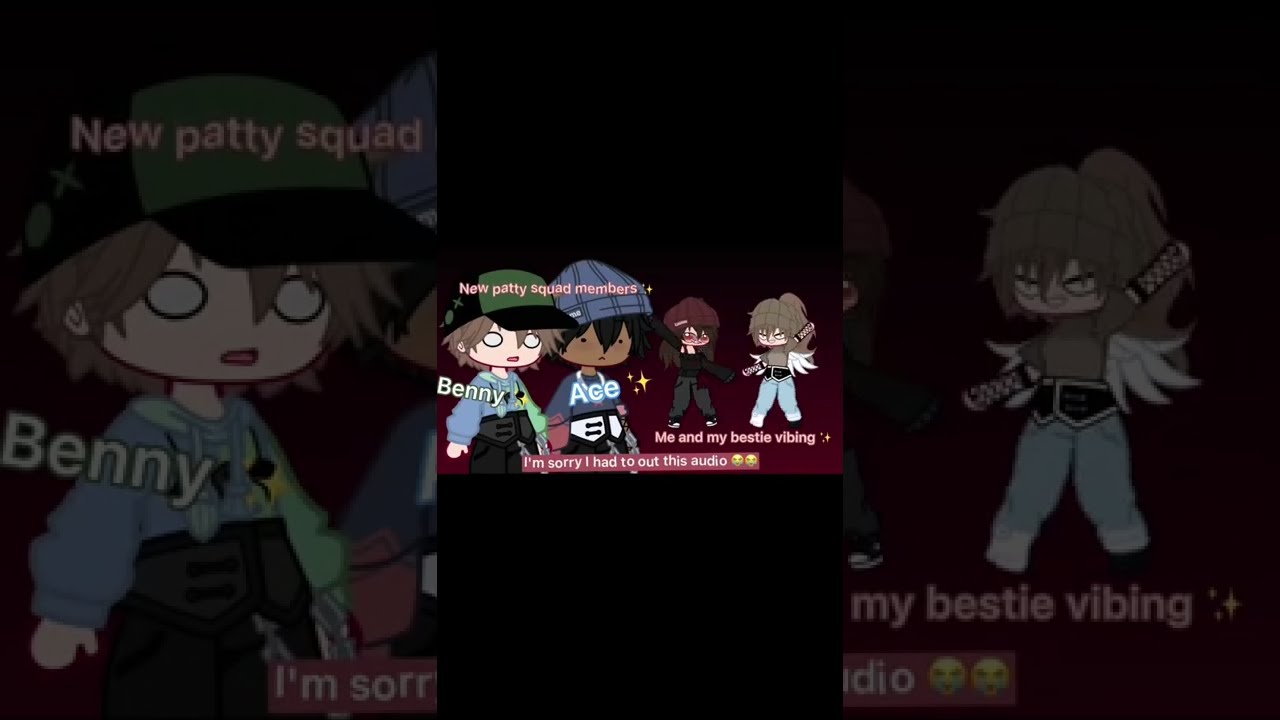The image is divided into three vertical sections. The central section features a pink background with four cartoon characters. The text above them reads "New Petty Squad members Benny and Ace." Benny is depicted as a character with shaggy, light brown hair, a black and green hat, completely white eyes outlined in black, and a blue and green shirt. Next to him is Ace, a dark-skinned character with a blue hat and hair covering his face. Flanking these two characters are two others with mostly obscured features. The text over the image includes "me and my bestie vibing" and "I'm sorry I had to cut out the audio." Each side section contains a darkened, close-up version of the respective characters from the middle section. The image is bordered at the top and bottom with black strips.